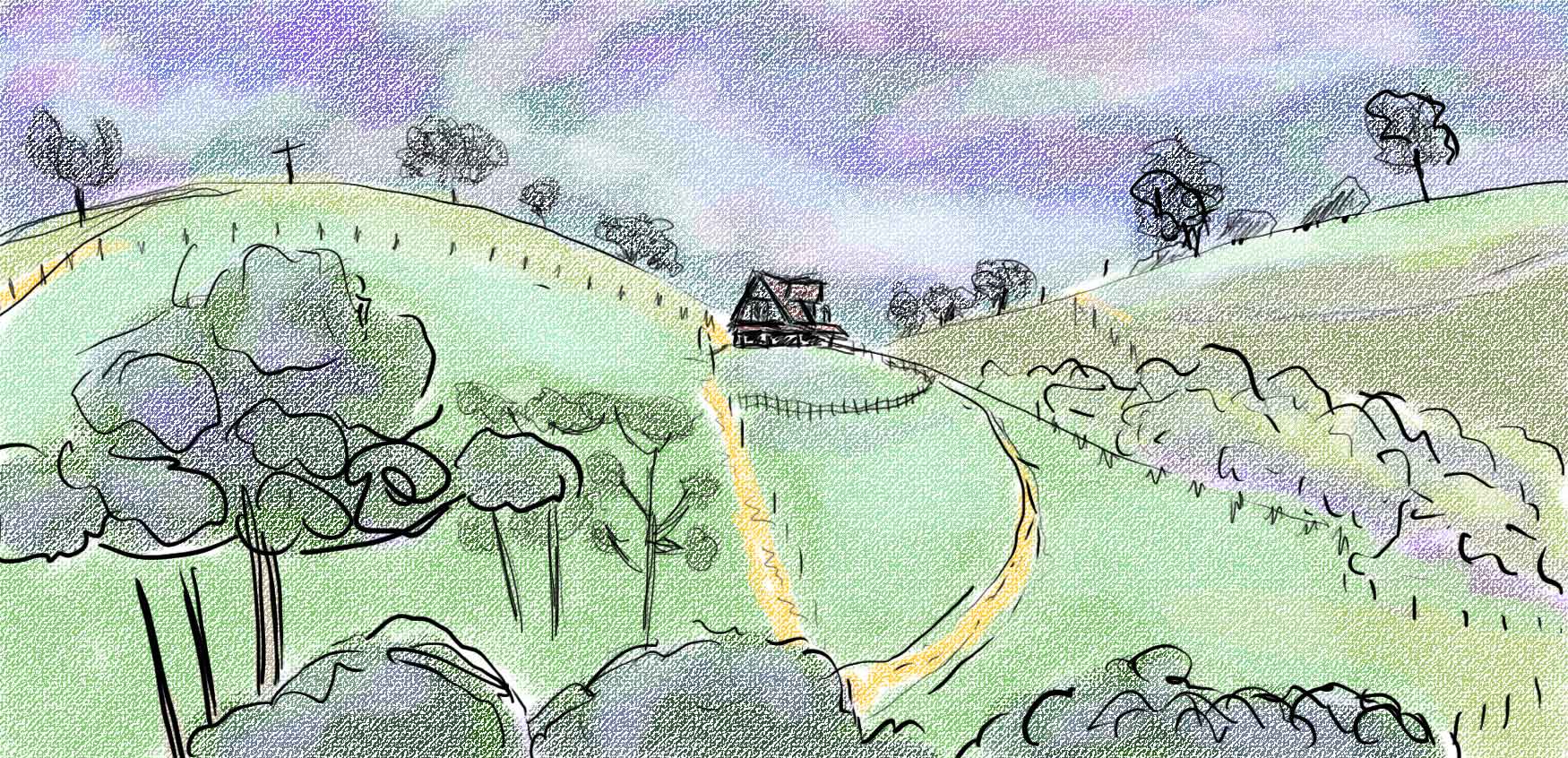This colored pencil and watercolor artwork on canvas depicts a vibrant countryside landscape with various intricate details. In the foreground, there are tall trees with black branches, their leaves a mix of deep green and purple. The middle ground showcases rolling green hills and valleys interspersed with yellow dirt pathways that weave through the scene. A house, reminiscent of a farmhouse, sits perched on one of the hills, surrounded by a slightly visible fence. Scattered around are bushes and markings that resemble a rustic fence, enhancing the rural charm. The background features more hills, which blend hues of green and purple, and the entire scene is set beneath a sky that shifts through a cotton candy spectrum of purple, light blue, pink, and white. This vivid blend of colors and the intricate pen or pencil outlines give the piece a dynamic and textured feel, drawing the viewer's eye from the detailed foreground to the softer, dreamy horizon.